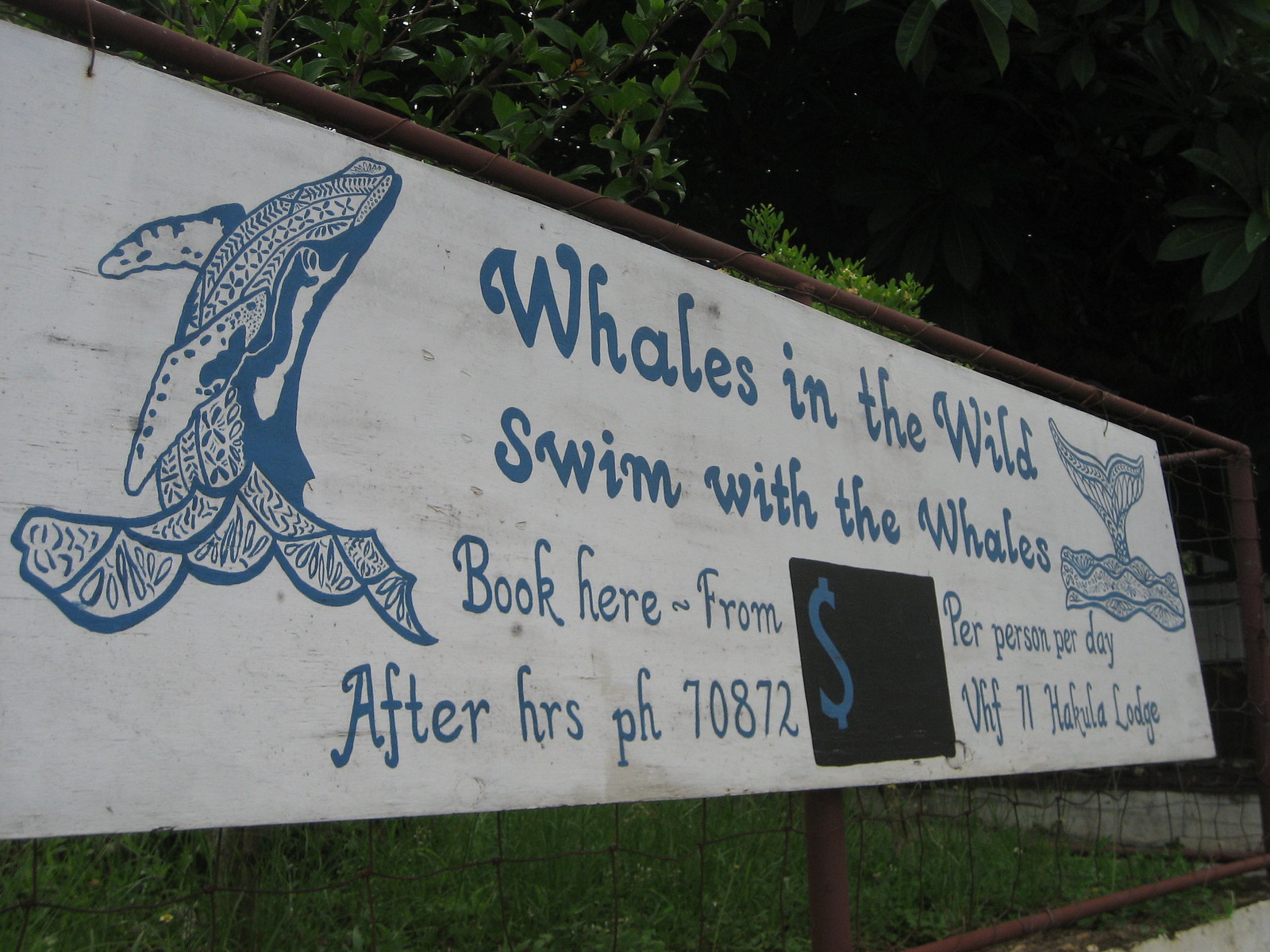A white wooden sign with blue text is attached to an old, rusted brown fence, surrounded by green vegetation including grass, vines, and trees. The large sign, featuring tribal-style illustrations of a breaching whale on the left and a whale tail above the water on the right, reads: "Whales in the Wild, swim with the whales. Book here from [blank], per person per day. After hours, PH 708-872, VHF-71, Hakuna Lodge."